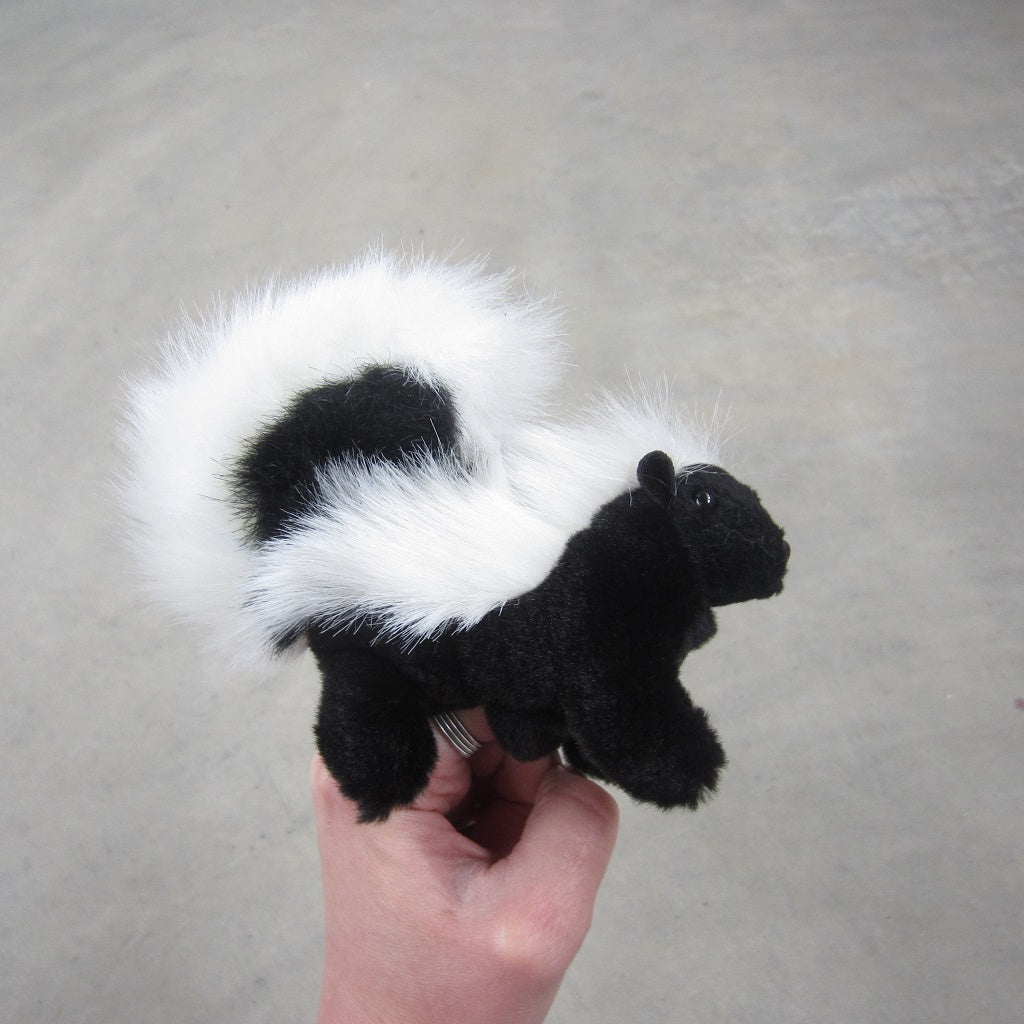In this photograph, an older-looking human hand is holding a small plush toy skunk. The hand is positioned with the index finger extended and the rest of the fingers curled into a fist. The person is wearing a distinctive silver ring on their index finger, which consists of four closely connected silver bands. Mounted on the extended index finger is the plush skunk, giving it the appearance of a finger puppet. The toy skunk is predominantly black with characteristic white fur running along the top of its head, down its back, and on the edge of its upward-curled tail. The skunk features a black plastic eye and small black ears. The background of the image resembles a gray laminate surface, creating a neutral backdrop that highlights the details of both the hand and the plush toy.